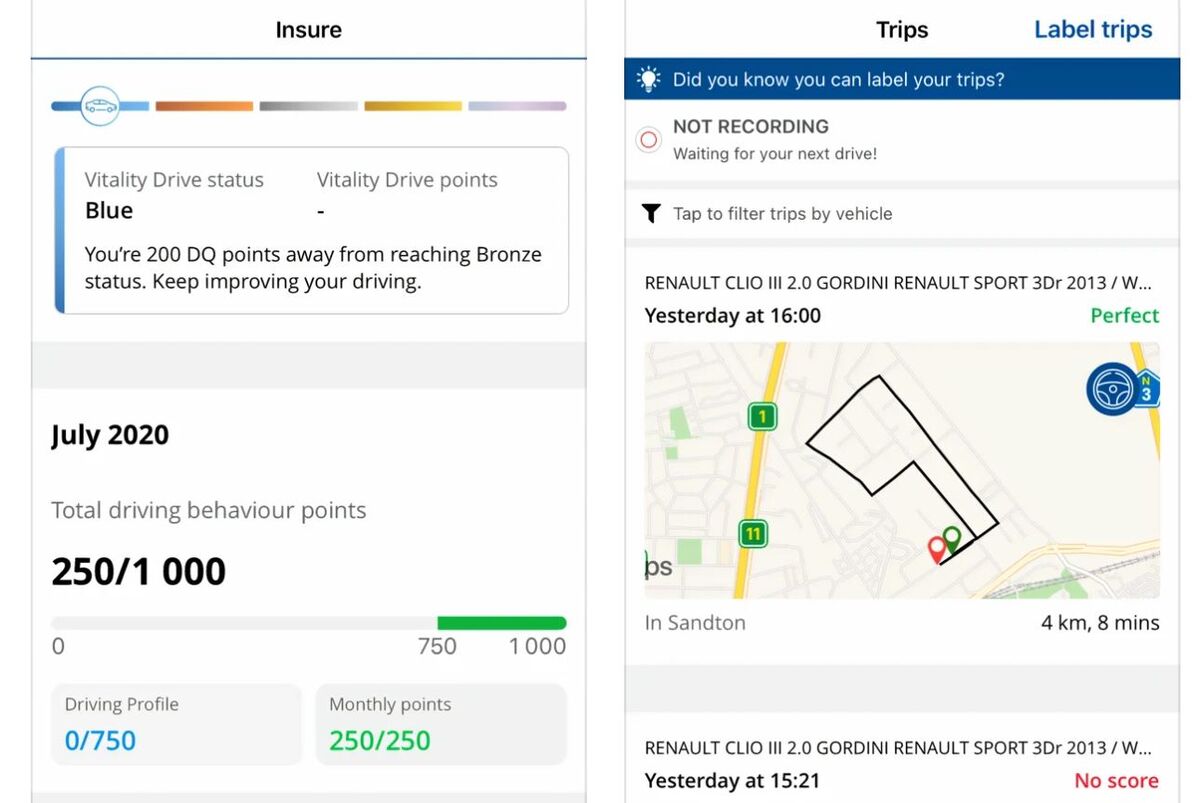**Caption:**

The screenshots display details related to driving insurance and driving behavior monitoring. The first screenshot shows an app interface with 'Insure' at the top. Below that, there's a visual representation featuring a car on a teal line followed by orange, varying shades of gray, yellow, and purple lines. The interface specifies the 'Vitality Drive Status' as blue with no 'Vitality Drive Points' recorded. It mentions that the user needs 200 DQ points to reach bronze status and encourages improving driving habits. For July 2020, the user has a total of 250 out of 1,000 driving behavior points, zero points for their driving profile out of 750, but full monthly points of 250 out of 250.

The second screenshot shows the 'Trips' section, starting with a blue-labeled prompt saying, "Did you know you can label your trips?" followed by a status message "Not recording, waiting for your next drive." There is an option to filter trips by vehicle. Listed is a 'Renault Clio 3, 2.0, Gordini Renault Sport', with the last trip recorded at 'San Tan' yesterday at 16:00 for 4 kilometers over 8 minutes with a "perfect" score. Another entry for the same vehicle, yesterday at 15:21, shows no score, highlighted in red.